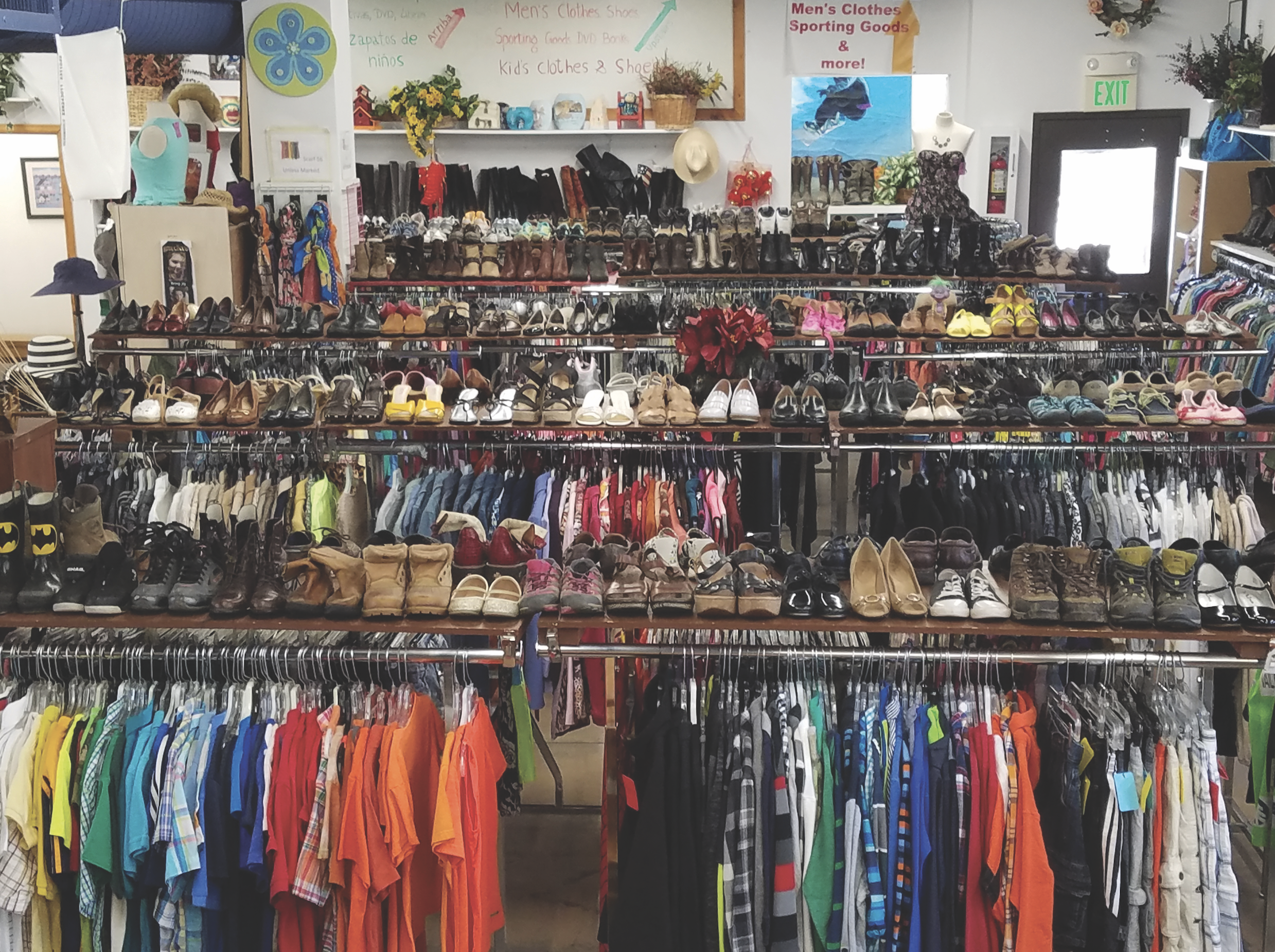This detailed image captures the bustling interior of a thrift or second-hand store, reminiscent of a Goodwill. The scene includes several rows of clothing racks, each adorned with a silver metal bar that supports a diverse collection of brightly colored clothing, ranging from men's t-shirts in the foreground to various women's garments towards the back. Each rack is topped with a flat brown wooden shelf laden with shoes, organized by type — men's boots, women's shoes, and children's footwear among others. The back wall of the store is white and features multiple signs, including a whiteboard listing categories such as men's clothes, shoes, sporting goods, D&D boots, and kids' clothes. Additionally, a prominent red-text sign directs customers to Men's Clothes, Sporting Goods, and More. A well-lit exit door with a clear sign above it is visible to the right. The clothes on the nearest rack appear arranged in a vibrant, somewhat rainbow order from yellow to black, interspersed with patterned pieces and pants towards the end.